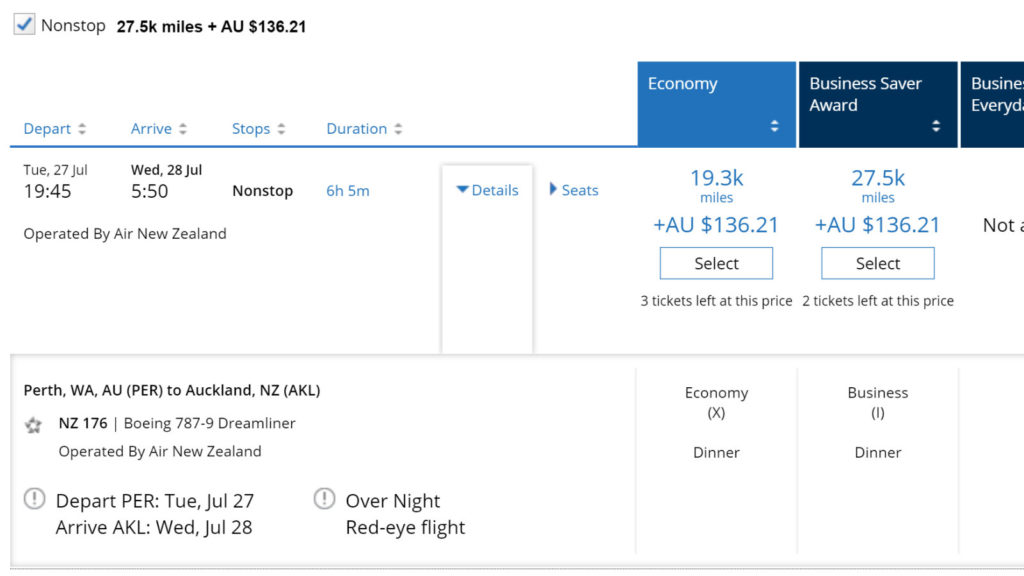The image displays a flight booking detail. At the top, there is a highlighted box with a checkmark indicating the selected option: “Non-stop, 27.5 kmiles plus AU $1.00, and AU $136.21”. Below this, there are columns labeled “Depart”, “Arrive”, “Stops”, and “Duration”. Under the “Depart” column, it specifies “Tuesday, 27 July 1945”. Under “Arrive”, it states “Wednesday, 28 July 540”. The “Stops” column confirms “Non-stop” and the "Duration" column shows “6 hours and 5 minutes”. To the side, there are boxes: a blue one labeled “Economy”, a darker blue one labeled “Business Saver Award”, and another labeled “Business Every Day”.

Further details are provided:
- Under “Economy”, it notes "19.3 kmiles plus AU $136.21" and includes a "Select" button, alongside a note that says "3 tickets left at this price."
- Under the “Business Saver Award” column, it shows "27.5 kmiles plus AU $136.21". 

Additionally, there are buttons marked “Details” and “Cease” for further options.